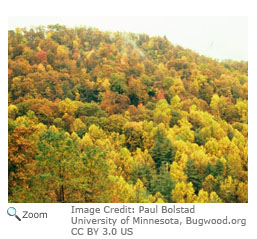The image is a detailed photograph of a tree-covered hillside displaying a stunning array of autumnal colors. The vibrant foliage includes hues of yellow, light brown, orange, green, and a few red trees, forming a densely packed canopy with just the tree tops visible, creating a clustered mosaic of colors. A whitish-blue sky forms the backdrop, adding depth to the scene. A subtle white area in the center of the photograph hints at a possible waterfall, though it's not clearly defined. Beneath the image, in the bottom left corner, there's a small magnifying glass icon labeled "Zoom," and to its right, the text reads, "Image Credit: Paul Bolstad, University of Minnesota, bugwood.org, CC BY 3.0 US." This image appears to be a screen grab from a website, capturing a picturesque moment of seasonal transformation in the forest.